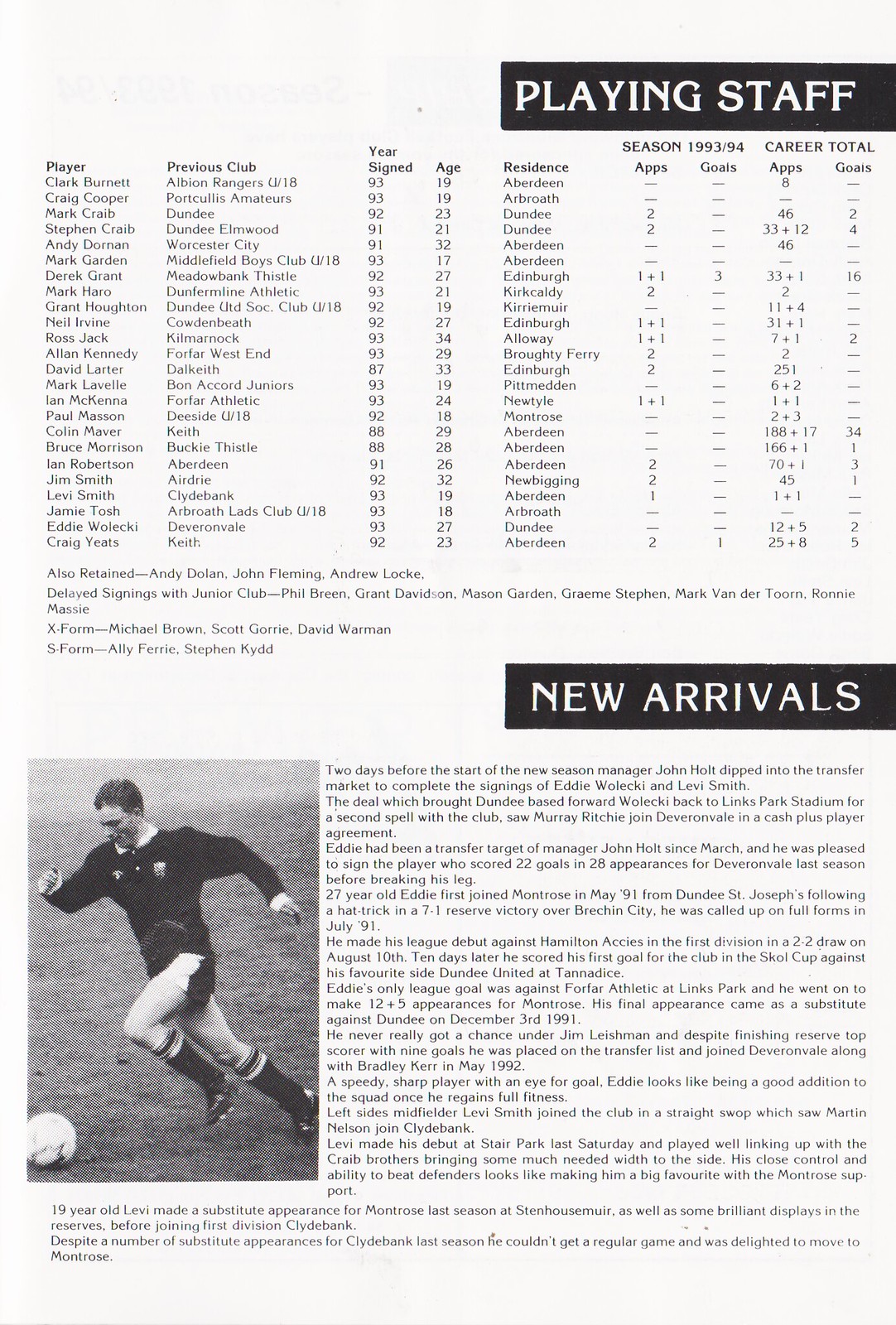The image is a page from an old sports booklet or newspaper, printed in black and white, with a layout reminiscent of earlier decades. In the top right corner, a black rectangle with bold white letters reads "Playing Staff." Below this section, there is a detailed list that includes columns titled "Player," "Previous Club," "Year Signed," "Age," "Residents," "Season 93/94," and "Career Total Apps Goals." This meticulously lists numerous players, their respective details, and statistics in a grid format.

Further down the page, another black rectangle with bold white letters marks the section "New Arrivals." Underneath, there is a block of text providing explanations or descriptions related to the new arrivals mentioned. On the left side of the page, there is a black and white photograph capturing a moment from a soccer match: a player, dressed in a black uniform, is poised to kick the ball, exuding focus and intensity. The photo, rendered in shades of gray, black, and white with a silver-tone quality, amplifies the nostalgic feel of the entire page.